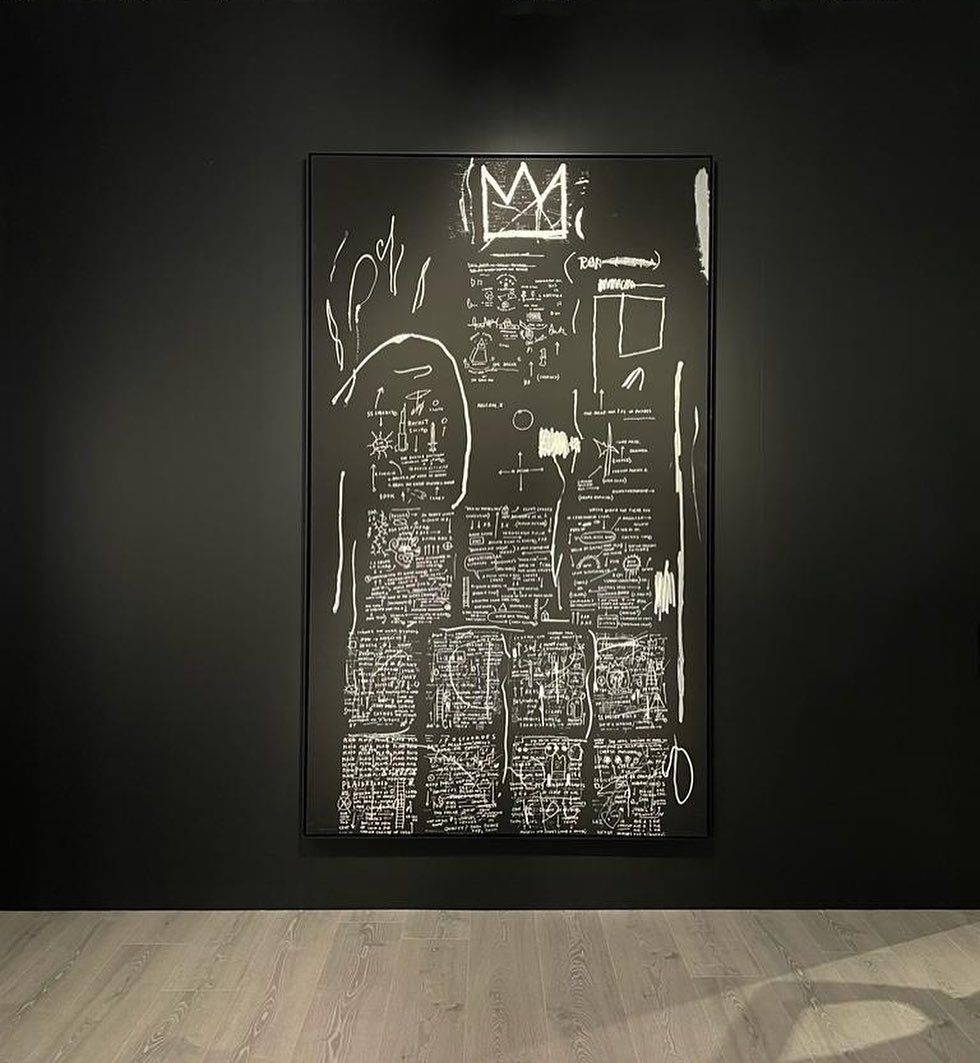In the image, we see a large, rectangular painting, possibly a canvas, hanging on a black-collared wall, suggesting it may be in an art museum. The painting, framed by a thin black border, features an entirely black background covered with various white scribbles, symbols, and unreadable text. At the top of the canvas, there is a rough, outlined drawing of a crown. The wall against which it hangs contrasts with the wooden floor below, which is neither too dark nor too light. The painting is illuminated by lights shining up from below, adding to the setting's gallery-like ambiance. Overall, the artwork’s chaotic text and imagery, combined with its prominent crown symbol, create a striking visual display.